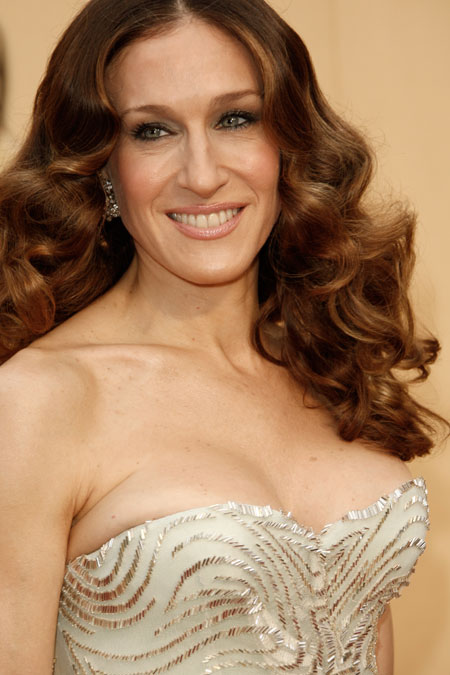The image features actress Sarah Jessica Parker, elegantly dressed, possibly for an awards ceremony. She is wearing a strapless, light champagne-colored dress adorned with darker golden copper trim and intricate silver beadwork. Her attire suggests the event is formal and prestigious. Sarah Jessica Parker, an older yet strikingly beautiful woman, has light skin and a graceful appearance. Her chestnut-reddish brown hair is long, floofy, and curly, parted in the middle, and styled to be voluminous. She has light-colored eyes, perhaps bluish-green, and her makeup is tasteful with light pink, shiny lipstick. A shiny earring is visible on her right ear. She is smiling warmly, showing her teeth, and glancing over her right shoulder, which appears as the left side of the photo. The background is a light peachy tan, providing a subtle backdrop that accentuates her presence. The photograph, a close-up from the ribcage up, captures her poised and radiant demeanor effectively.